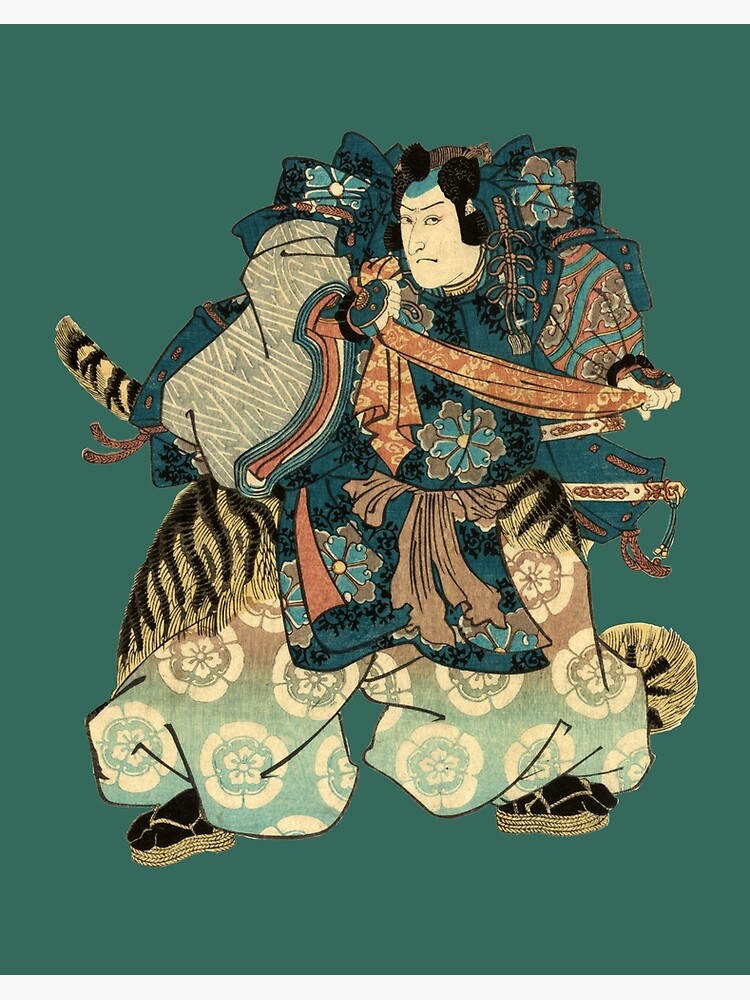The image depicts a detailed, painting-like illustration of a figure that blends elements of Chinese and Japanese traditional attire, with a strong emphasis on intricate details and vibrant colors. The backdrop is a rich, alpine green, providing a dark and verdant setting for the scene. Central to the image is a figure dressed in ceremonial regalia with floral patterns adorning their flowing capes. The figure's black hair is styled into several buns, and they wear a distinctive headdress. Their attire includes very baggy clothes and pants, combined with unique rope-like sandals. The individual is seen holding a material that extends from one hand to the other, draping slightly on the left side. Behind the figure, two swords are partially visible, tucked into their waistband, adding to the samurai-esque appearance. The major colors in the image include shades of blue, brown, cream, yellow, black, and white, all intricately woven into the composition to create a harmonious and captivating visual experience.